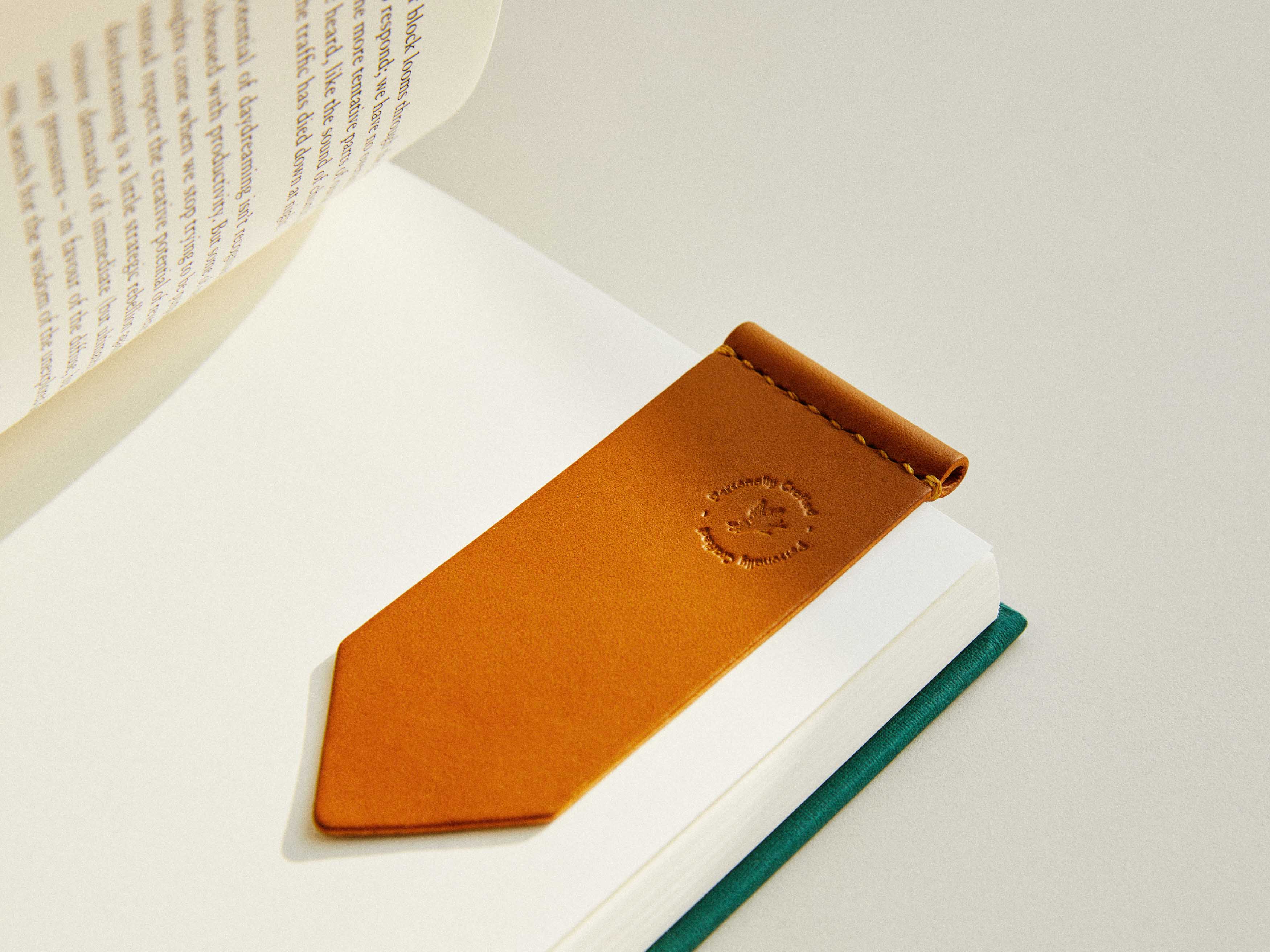The image depicts a close-up, daytime indoor shot of a hardcover book that is partially open, laying on a beige surface. The hardcover of the book is green. The left-hand page is folded over and filled with black font writing, while the right-hand page is blank. Resting on the blank page is a light brown leather bookmark, intricately stitched and shaped like a tie with a diamond-shaped end. The bookmark features the word "certified" stamped or etched into the leather and has a circular piece protruding from the end, laying flat within the book, keeping the reader’s place.